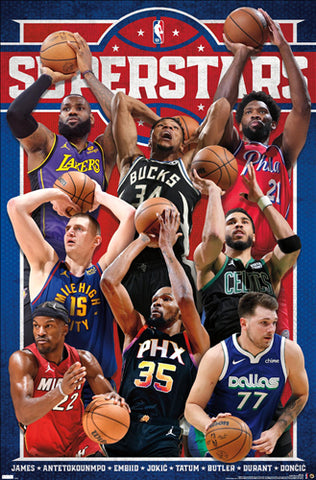This vertically oriented poster, perfect for hanging on your wall, showcases eight NBA superstars against a striking blue background. The standout title "Superstars" is emblazoned in bold white letters on a red rectangle near the top, accompanied by the iconic NBA logo featuring Jerry West's silhouette in red, white, and blue. The poster is divided into three tiers: three players at the top, two in the middle, and three at the bottom. The players, depicted in dynamic poses holding basketballs, are from various NBA teams including the Lakers, Phoenix, and Dallas. Notable athletes like LeBron James, who appears in the top left with an arm sleeve, are among those featured. The bottom section of the poster lists the players' last names, which include James, Antetokounmpo, Embiid, Jokic, Tatum, Butler, Durant, and Dončić. The vivid imagery and layout make this a compelling piece for any basketball fan.